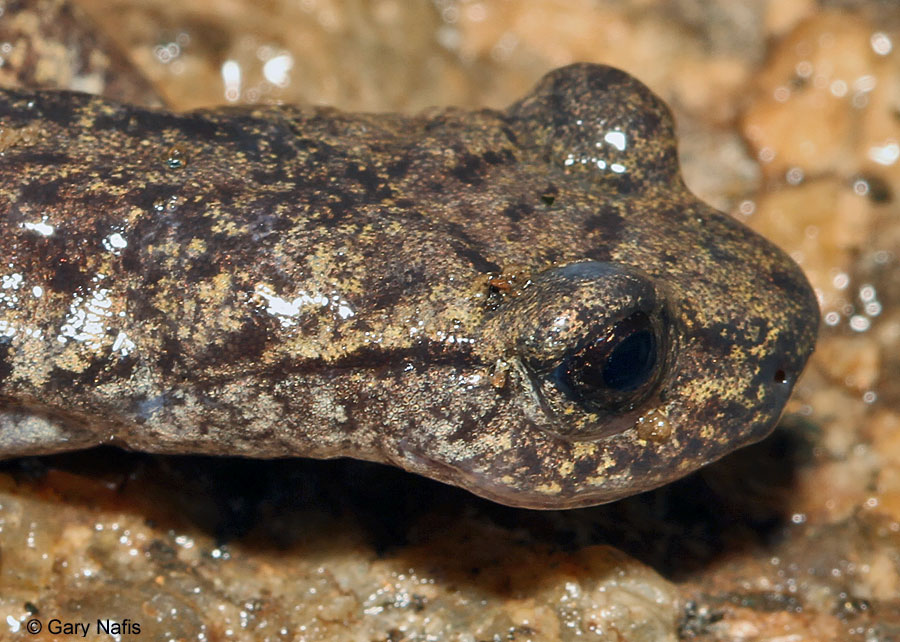This highly detailed, close-up photographic image captures the head and neck of a reptilian or amphibious creature, likely a lizard with gecko-like features. The animal's rounded nose and bulbous, black eyes, set on the sides of its head, are prominent. Facing right, the creature's head and part of its neck are the central focus. The skin, covered with black and white speckles, appears shiny and wet, reflecting the camera's flash, giving it a slimy texture. The neck curves slightly back to the left and is primarily brown with scattered light and dark spots. The surface beneath the animal resembles glistening brown marble, featuring hues of white and orange with a slightly gooey appearance. In the bottom left-hand corner of the image, the text "C. Gary Nafis" is clearly visible, adding a finishing touch to the photograph.